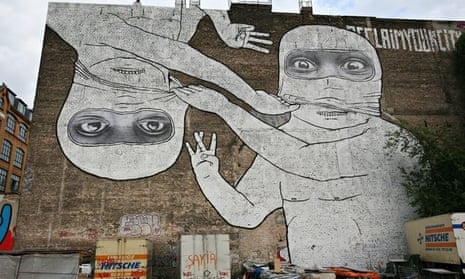The image captures a detailed mural on the side of a tall, weathered, grayish-white brick building, which appears very old and somewhat dirty. The mural spans the entire height of the building, depicting two lifelike figures rendered entirely in white. Both figures are engaging in the act of pulling masks off each other’s faces. The figure on the left is upside down, hovering adjacent to the upright figure on the right. Each figure is shirtless and only reveals their eyes and the bridge of their nose, with the masks being peeled back to expose their mouths. The eyes of the figures are strikingly realistic, resembling actual photographs. Below the mural, scattered containers and the backs of semi-trailers and large box trucks create a cluttered scene. At the top left corner of the building, the words "Reclaim Your City" are painted in white, against a backdrop of blue and white sky peeking through.